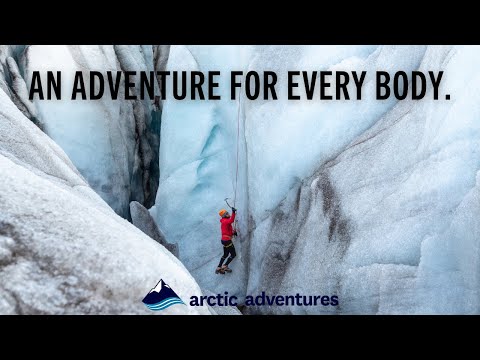The image is a detailed poster advertising "Arctic Adventures." It features a striking visual of a hiker dressed in a red-orange coat and black pants, scaling an imposing vertical wall of ice in an icy, mountainous landscape. The hiker is equipped with an ice pick and secured by a rope that wraps around their waist and upper thighs, extending out of the frame to convey the challenging nature of the climb. Above the hiker, the words "An Adventure for Every Body" cleverly emphasize both the inclusivity and the physical demands of the activity. The text is divided to create a double entendre, highlighting both "everybody" and "every body." The scene is framed by black bands at the top and bottom of the image, adding to its dramatic effect.

At the bottom of the image lies the text "Arctic Adventures" in indigo, serif typewriter-style font, accompanied by a logo. The logo features a white mountain peak with a turquoise base, and a blue and white swoosh or wave-like element beneath it. An additional detail includes a small insignia of a mountain to the left of the text, enhancing the adventurous allure of the poster. The visuals are accentuated by the glacier's turquoise and smoky black hues, bolstering the overall aesthetic appeal and sense of exploration.